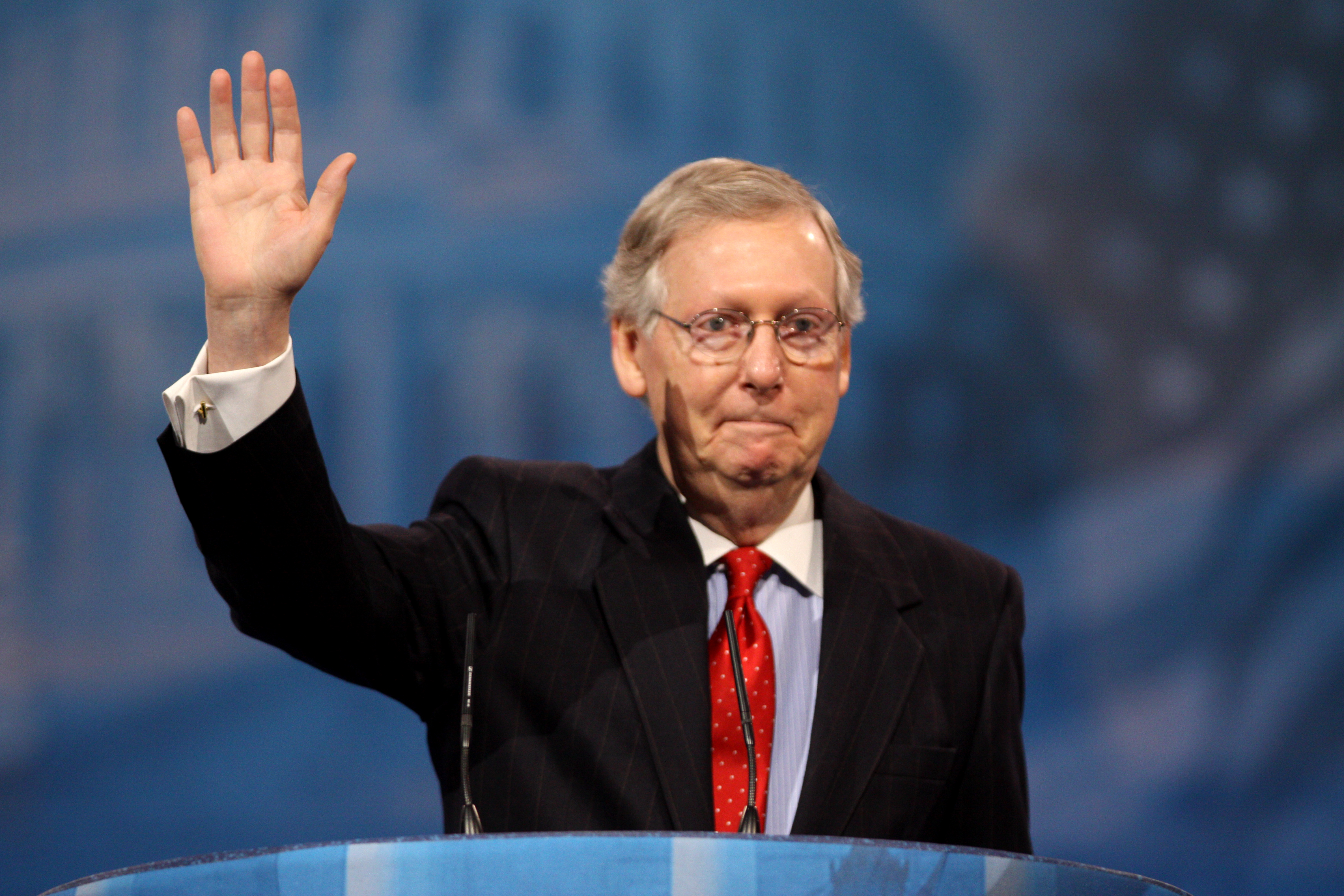The image is of Mitch McConnell, a seasoned politician, captured at an unmarked political event, presumably a debate or speaking engagement. He stands at a blue podium equipped with two small microphones at chest level. McConnell, with his gray hair neatly parted to the side, is wearing eyeglasses. His attire consists of a dark gray, almost black suit jacket with light gray vertical stripes, a light blue shirt with a white collar, and a red tie adorned with white polka dots. With a serious expression on his face, he raises his right hand in a waving gesture. The backdrop is predominantly blue, featuring blurred elements that hint at an American flag and possibly the Congress building, contributing to a patriotic theme. The color scheme in the image includes various shades of blue, red, white, black, and gray, indicating a professionally taken photograph with a focus on McConnell amidst a nondescript setting.